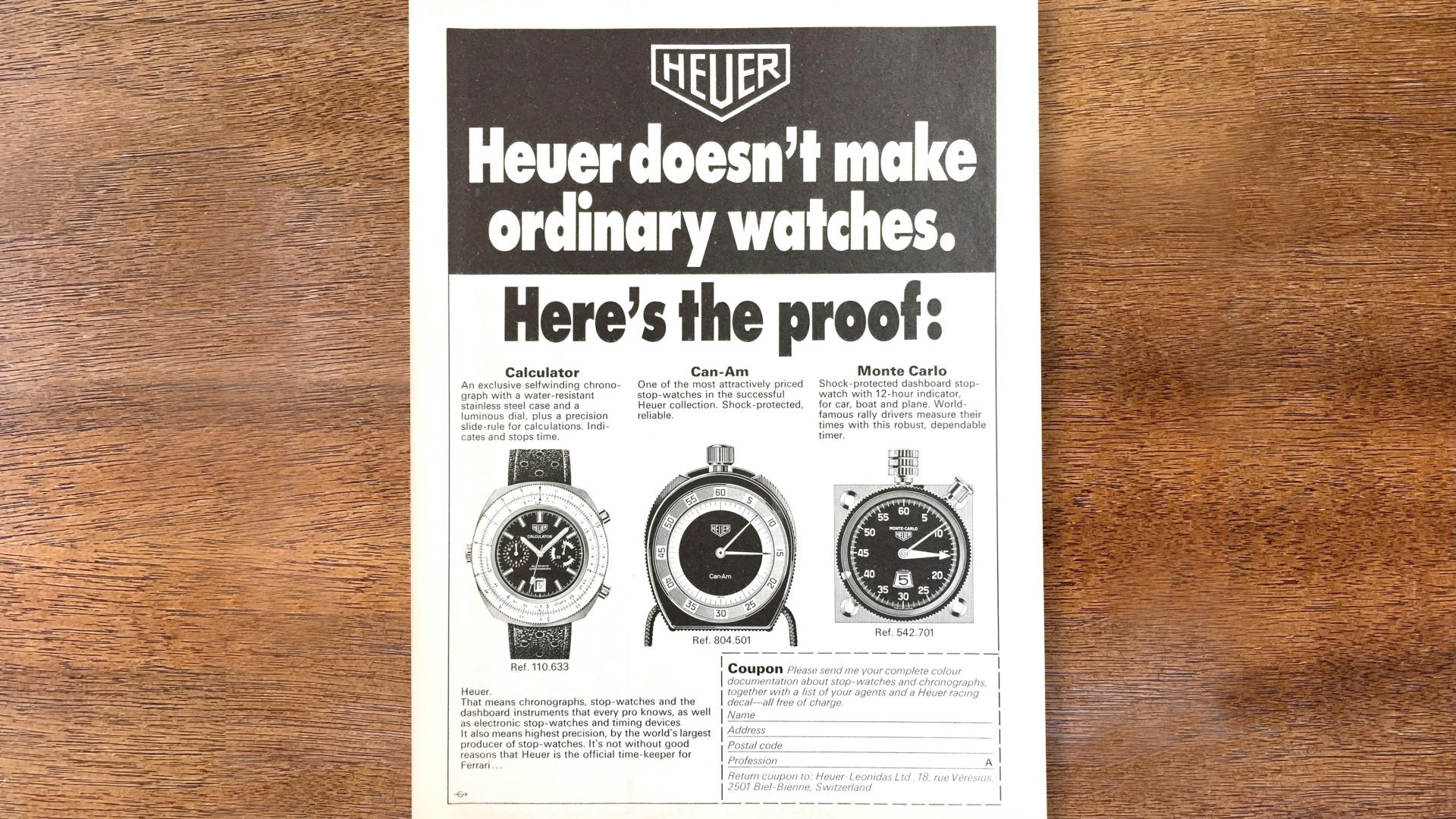This black-and-white newspaper advertisement for Heuer watches is placed on a wooden table. At the top, the Heuer logo, which is enclosed in a home plate-shaped symbol, prominently features white bold text declaring, "HEUER DOESN'T MAKE ORDINARY WATCHES." Below, in large black text, it announces, "HERE'S THE PROOF:" followed by three distinct sections, each showcasing a different watch model. The first section, labeled "Calculator", displays a Heuer watch with an attached leather band. The second section, "Can-Am", appears slightly blurred but shows a side view of a watch, featuring a noticeable knob on the top. The third section, "Monte Carlo", reveals a stopwatch-like timepiece with a similar top knob. Each section includes detailed text descriptions beneath the images. A paragraph of additional information is seen in the lower left corner, and a coupon with dashed lines, requiring personal details like name and address, is situated in the lower right corner.